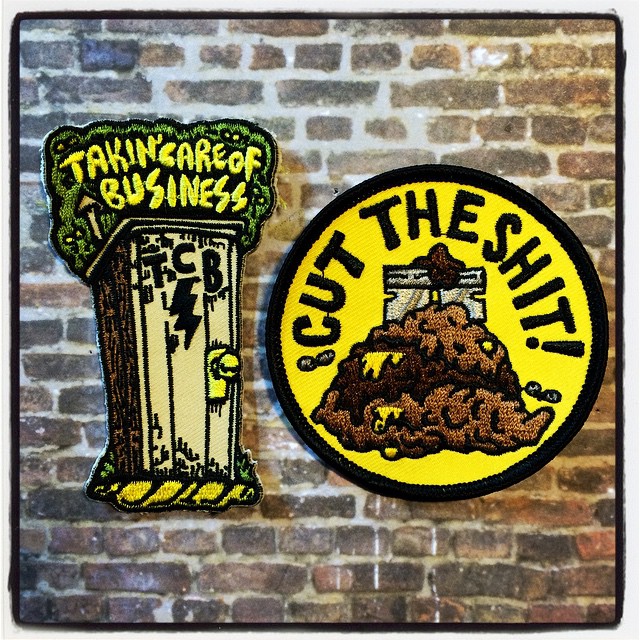The image depicts two detailed fabric patches set against a textured brick wall with a simplistic black border framing the scene. The bricks vary in shades of gray, brown, black, tan, and reddish hues, and are held together with white mortar. The patches are prominently positioned in the center of the image.

The left patch features a rectangular design with an outhouse illustration. The top of the patch has a black background with yellow text that reads "Taking Care of Business," and beneath it is an outhouse depicted in brown wood, with green trees around it. The center of the outhouse door is adorned with a golden handle and a yellow outline. Below the outhouse, the letters "TCB" with a black lightning bolt beneath it are prominently displayed.

The right patch is circular with a yellow background and black text circling the top, exclaiming "Cut the Shit!" At the center of this patch, a silver razor blade cuts through a brown mound, representing feces, from which yellowish material is seen emerging. The patch also features small fly-like ovals with wings flanking the sides of the mound.

The scene, potentially set outdoors in the middle of the day, gives an impression of being against the side of a building, where the vibrant colors and intricate details of the patches contrast sharply with the rustic brick background.